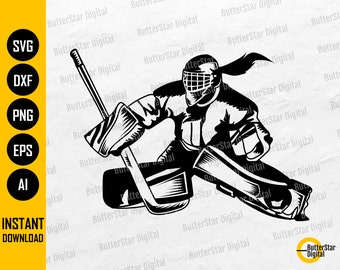The image depicts a detailed black-and-white drawing of a hockey goalie in a crouched position, ready to block incoming pucks with pads on his knees and a stick in his left hand. The goalie is likely female, as indicated by the long ponytail emerging from the back of the helmet, but this detail could be ambiguous. The helmet features a face guard for protection. The entire composition is set against a white background, featuring a gray watermark that reads "Butler Star Digital" in a repetitive pattern across the backdrop. On the left side of the image, there is a vertical yellow bar with five black circles, each containing white text that lists file formats: SVG, DXF, PNG, EPS, and AI. Below these, in black text, the phrase "instant download" is clearly visible. In the bottom-right corner, there is a logo encased in a yellow circle that once again states "Butler Star Digital" in black text.